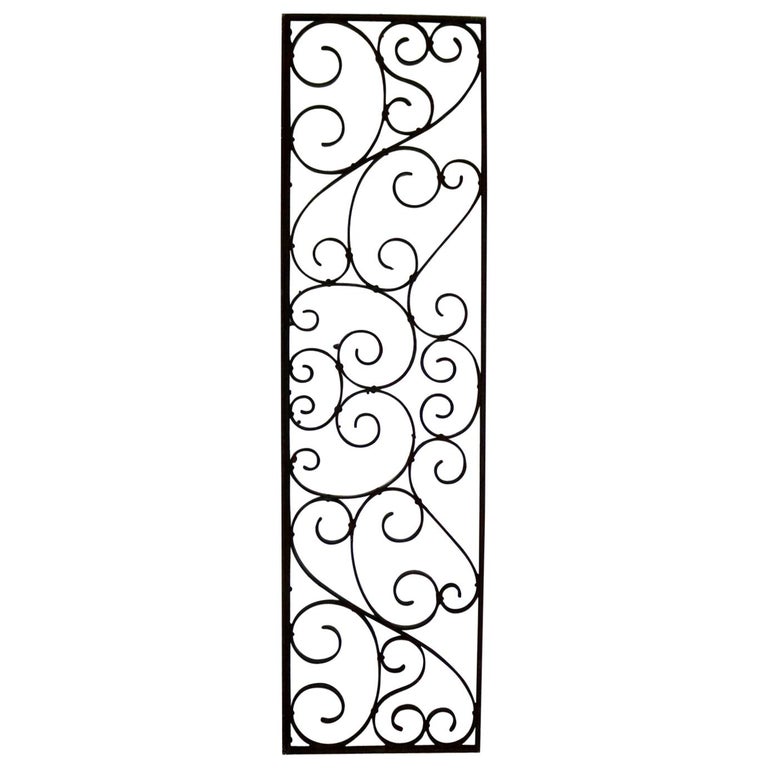The image depicts a tall, narrow, rectangular piece of black wrought iron decoration, with an overall width of approximately one to two feet. The wrought iron is meticulously crafted into an array of intricate patterns, predominantly featuring S-shaped and C-shaped curly-Qs. Some of these curves culminate in elegant heart shapes, especially near the top, and kidney-like forms as they converge towards the center. The decorative piece appears borderless on the outside but is framed all around by a thicker left side and uniformly thick top and bottom edges compared to the thinner right side. The design showcases a thoughtful arrangement, with inverted matching loops at the top and bottom, resembling elaborate spirals and arc shapes. The object evokes the aesthetic of wrought iron fencing, possibly serving as a decorative panel or frame, characterized by its cohesive and artistic spiral motifs soldered seamlessly into the upright frame, exuding an overall sense of ornamental craftsmanship. The background of the image is plain white, dotted sporadically, adding to the visual emphasis on the intricate ironwork.